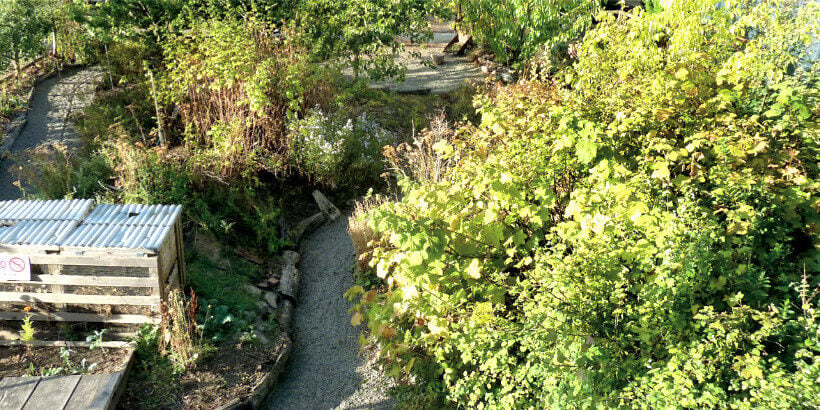The horizontal rectangular aerial photograph captures a vibrant outdoor scene bathed in natural light. Dominating the right side and the center of the image are dense, green leafy trees, alongside a stream meandering from the bottom of the frame and disappearing off to the right, obscured by the foliage. This waterway features a stony beach along one of its banks, suggesting a natural, slightly wild environment. The lower left corner showcases an intriguing four-story building with a distinctive roof, possibly surrounded by parking spaces, and brings a human-made element to the natural landscape. Additionally, nearby there is what appears to be a structure, possibly a deck or shed, adjacent to an organized area enclosed by wood and metal grating, hinting at either a pen for animals or a contained garden space. A small walkway winds through the lush greenery, providing a path through the otherwise overgrown vegetation. The image captures an idyllic, sunlit scene characterized by a rich palette of greens, browns, and grays, highlighting both the natural and constructed features in a bright and clear composition.